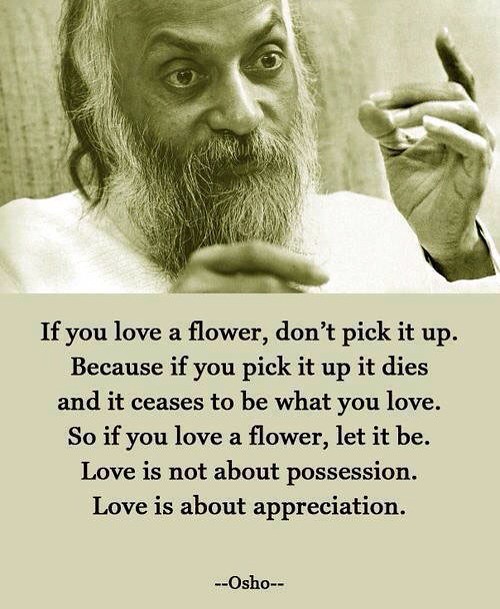The image showcases an inspirational poster featuring a notable quote attributed to Osho. The top half of the poster is a sepia-toned photograph of an older man with medium to long gray hair and a long gray beard. He appears to be in his 50s and is wearing a white garment. The man’s expressive face has raised eyebrows and wide-open eyes, and he is captured mid-gesture, with one hand partially raised and the other forming a gesture where his middle finger touches his thumb. Beneath the photograph, the background transitions to gray, displaying the quote: "If you love a flower, don't pick it up, because if you pick it up, it dies and it ceases to be what you love. So if you love a flower, let it be. Love is not about possession. Love is about appreciation." At the bottom of the poster, the name "Osho" is prominently written, framed by dashes on either side.